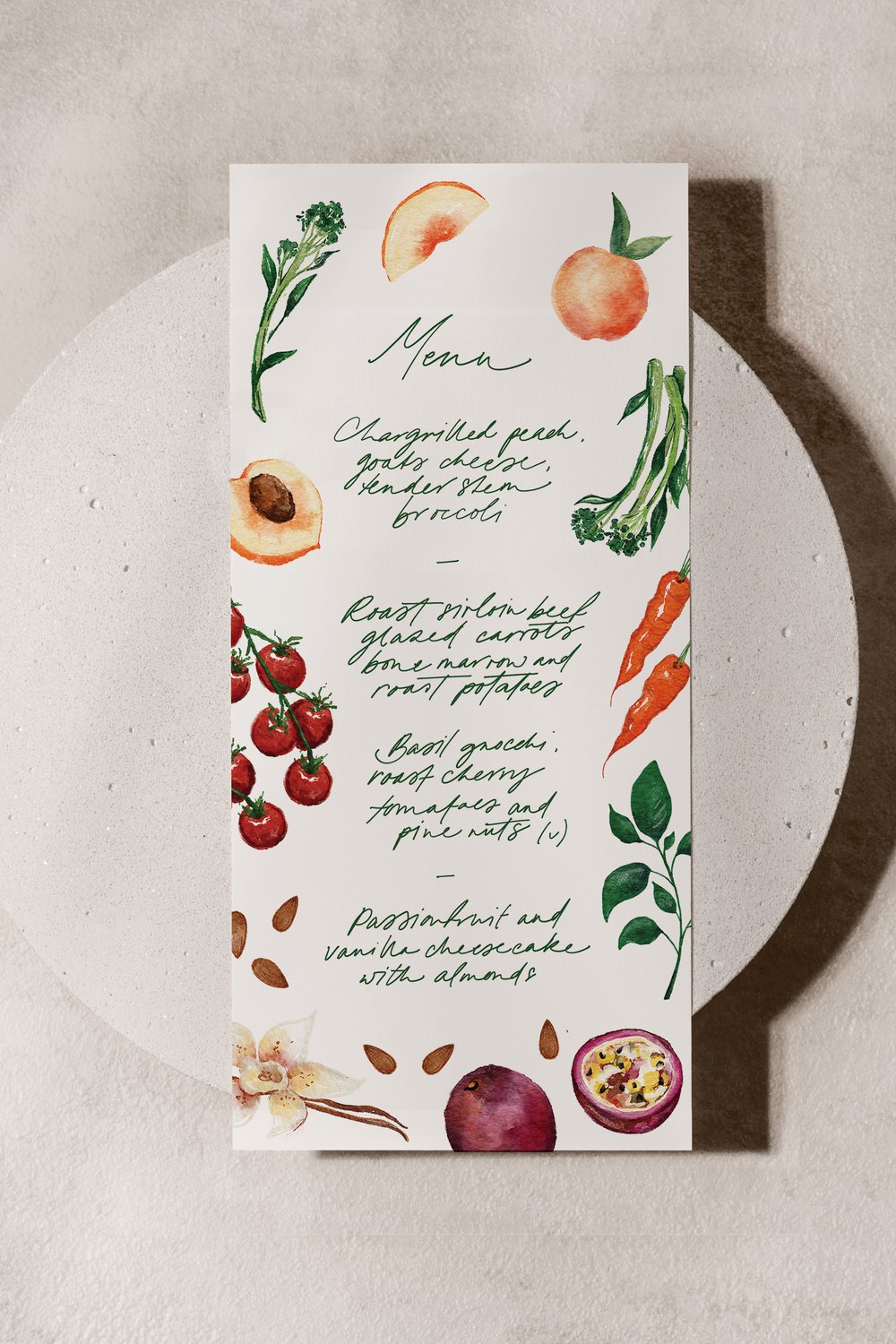This detailed portrait-oriented photograph showcases a rectangular menu card delicately placed atop a round, light gray stone slab, likely a raised clay plate, which casts a subtle shadow on the background. The menu card, executed in an off-white or white shade, is bordered with vibrant watercolor paintings of fruits and vegetables. Among the depicted items are sliced, halved, and whole peaches, broccolini, glazed carrots, cherry tomatoes, a vanilla bean, flowers, and passion fruits—one whole and one split open.

At the top of the menu card, written in a green, almost decipherable cursive script, the word "Menu" is prominently displayed. Below this heading, the menu items are listed:

1. Char-grilled peach, goat cheese, tender stem broccoli
2. Roast sirloin beef, glazed carrots, bone marrow, and roast potatoes
3. Basil gnocchi, roast cherry tomatoes, and pine nuts (marked with a "V" for vegetarian or vegan)
4. Passion fruit and vanilla cheesecake with almonds

The watercolors around the border directly correspond to the ingredients listed within the menu, creating a harmonious and visually appealing frame that ties the entire presentation together. The artistic renderings of the colorful ingredients echo the dishes and add an artistic flair to the otherwise simple design of the menu card.